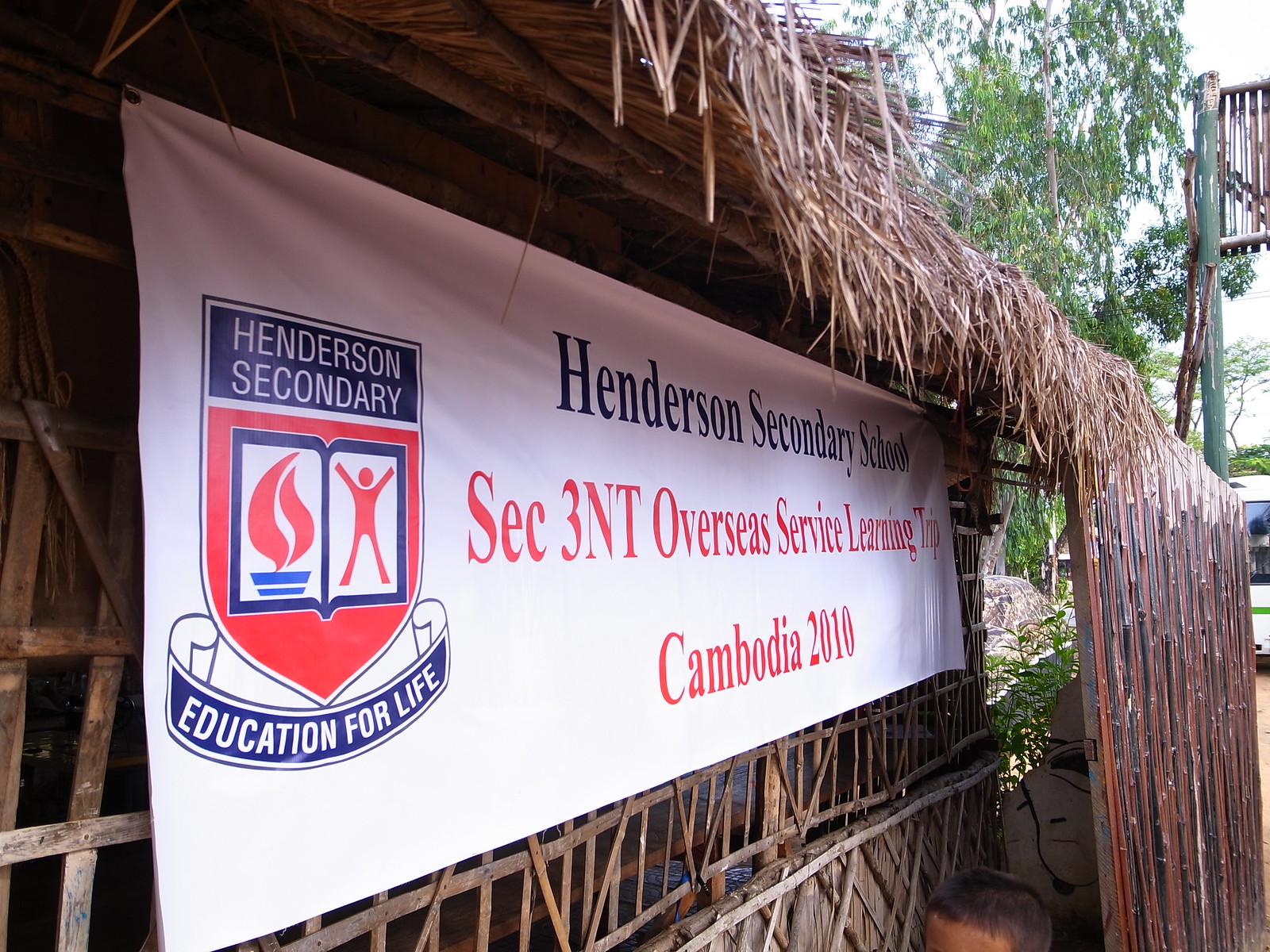In this image, we see a rustic building constructed from slatted wooden panels and topped with a straw thatch roof. Suspended diagonally across the front of the structure is a large, white rectangular banner. The banner prominently bears the text "Henderson Secondary School Section 3NT Overseas Service Learning Trip, Cambodia 2010." On the left-hand side of the banner, there is a detailed shield emblem. The top of the shield is blue with the text "Henderson Secondary," while the bottom is red featuring an open book, a stick figure with outstretched arms, and a red flame symbol. Below the shield, a blue ribbon banner reads "Education for Life." The banner hangs from the roof, below a thatched overhang, and in the backdrop, green trees add to the natural setting. The perspective of the photo is slightly angled, making the text somewhat challenging to read, and hints of additional structures, such as a platform with a railing, can be seen in the background. The scene is bathed in daylight.